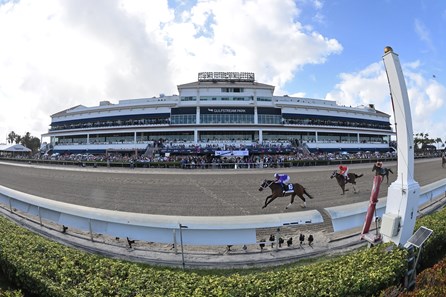The image captures a dynamic horse race, possibly near the photo finish line, taken with a fisheye lens that curves the elements in the frame. In the foreground, there is a grayish track bordered by whitish barriers resembling half walls, flanked by lush green grass. The racers are moving from the right; the lead jockey is dressed in blue, followed by another in red, while the rest are less distinct. To the far right stands a curved white pole, indicating the finish line. The background is dominated by a large, rectangular, white multi-level building with extensive seating and a windowed area at the top. Spectators can be seen outside, engrossed in the race. The sky is partly cloudy with light blue hues, suggesting a bright, sunny day. Overall, this detailed photograph offers a vivid portrayal of the intense, high-stakes moment at the race.